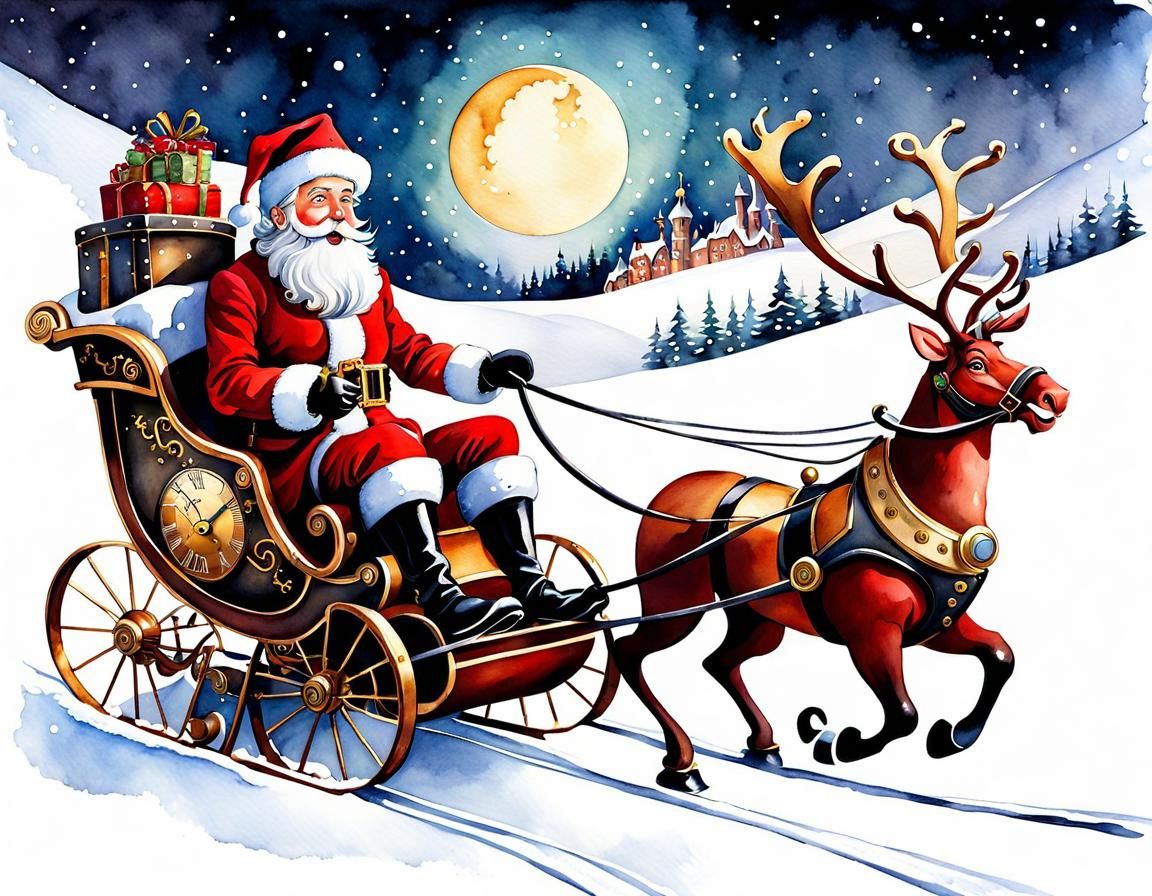The image depicts a vintage Christmas greeting card, featuring a winter landscape. In the foreground, Santa Claus sits in a traditional red sleigh, adorned with a clock, and pulled by a single reindeer. Santa, with his white beard, mustache, rosy cheeks, and wearing a red hat, jacket with white cuffs, black gloves, and black boots, holds the reins in his left hand. Behind him, a few presents are nestled in the sleigh. Under a yellow full moon, surrounded by stars in a dark night sky, Santa and his reindeer gallop over sloping, snow-covered hills dotted with pine trees. In the background, there's a castle-like building, possibly Santa's North Pole workshop, and some small homes peeking through the snowy landscape. The reindeer’s legs are mid-action, painting a vivid picture of movement as Santa journeys through the serene, snowy night.